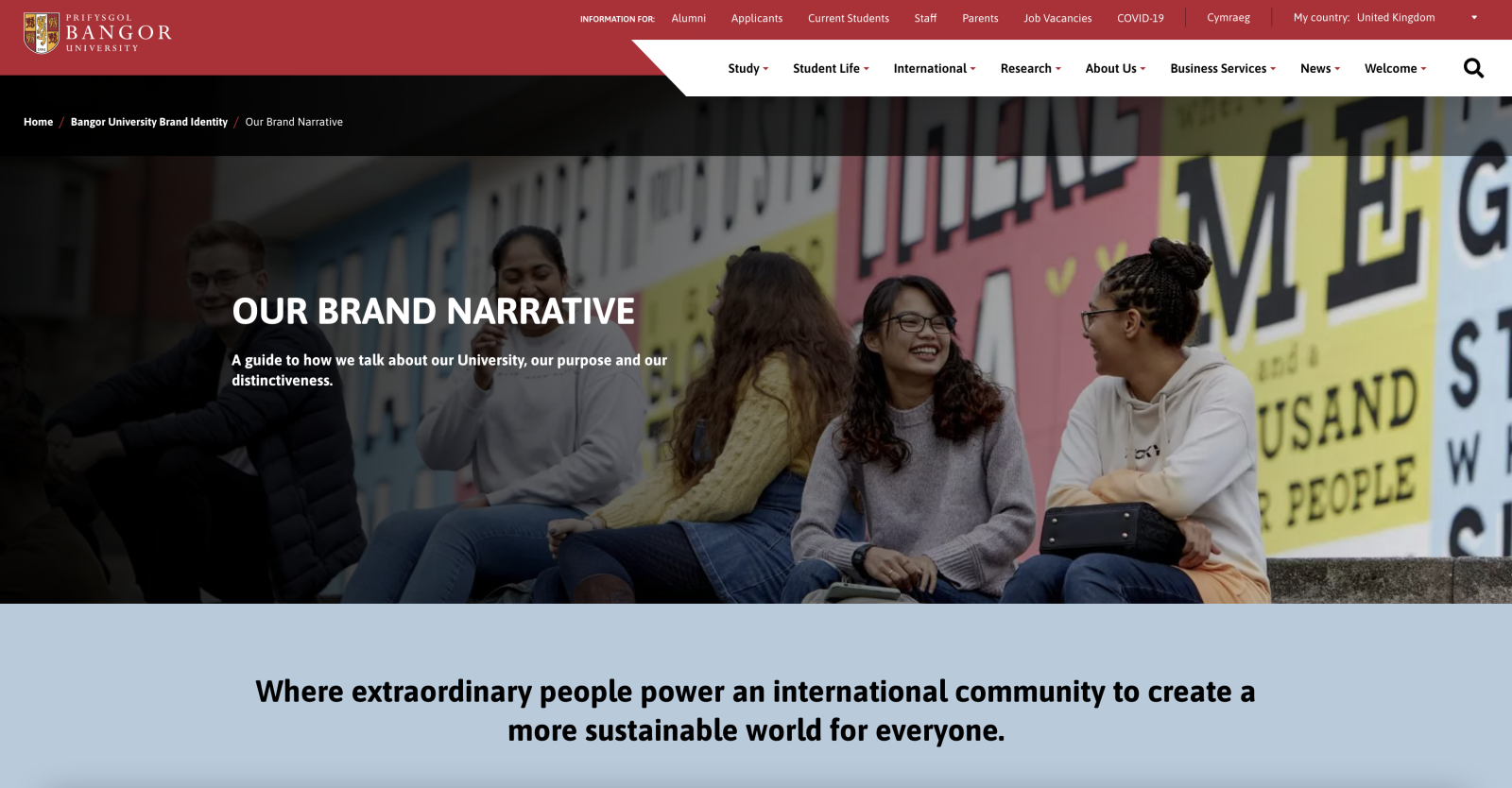The webpage of Bangor University proudly showcases a vibrant image of four female students seated on a ledge in front of a strikingly colorful sign brimming with letters. Two pairs of the girls engage in animated conversations with each other, while the one on the far left appears absorbed in a phone call. They all emanate happiness and camaraderie, contributing to a lively campus atmosphere.

Behind them, the colorful sign serves as both a visually captivating element and an informational display. Dominantly featured in the center is a white inscription detailing the university's brand narrative: "Our guide to how we talk about our university, our purpose, and our distinctions." Beneath this, a whitish-blue strip carries a profound message in black text: "Where ordinary people power an international community to create a more sustainable world for everyone."

At the top of the page, a navigation bar offers easy access to various sections, including "About Us," "International," "Research," and other essential categories, providing visitors with comprehensive information at their fingertips.